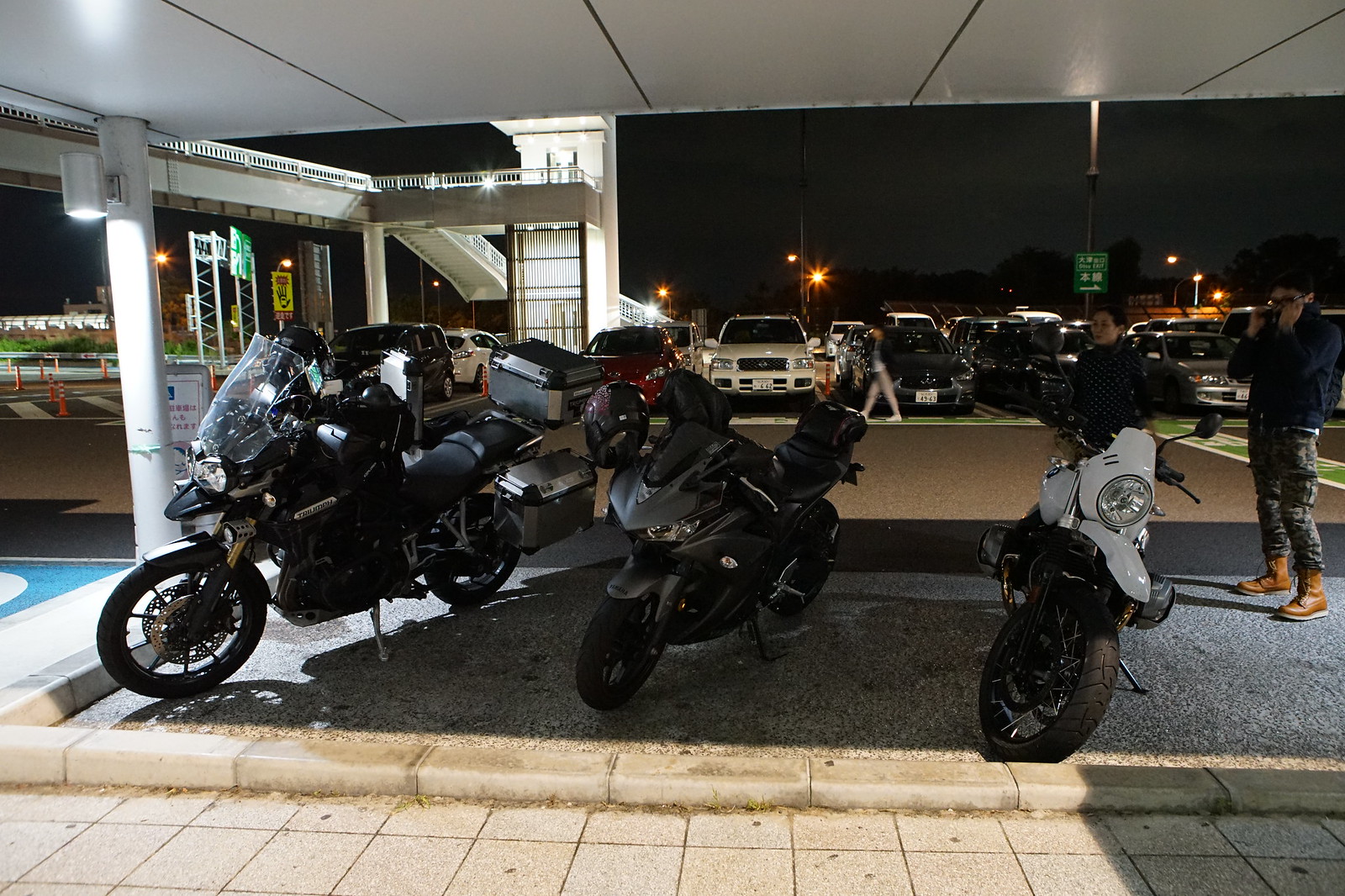In the foreground of this detailed nighttime photograph, three motorcycles are prominently parked on a gray gravel area adjacent to a walkway made of tan cement tiles. The first motorcycle on the right is white with black detailing, featuring a large round headlight and a white fender. The middle motorcycle, entirely black and gray, has a black helmet with purple trim hanging from one of its handlebars. The third motorcycle, positioned on the left, is also black and equipped with a see-through windshield as well as large storage boxes on the back. A white-skinned woman with dark hair and wearing a dark top stands next to the motorcycles. Next to her is a light-skinned man in a blue top, camouflage gray pants, brown boots, and glasses. In the background, out of focus, is a busy parking lot full of cars, with a person walking in front of them. Illuminated by streetlights, the setting includes an overhang supported by round pillars with can-shaped lights, adding a structured contrast to the parking lot scene. Additionally, a building and a small pedestrian bridge are visible towards the left side of the image.